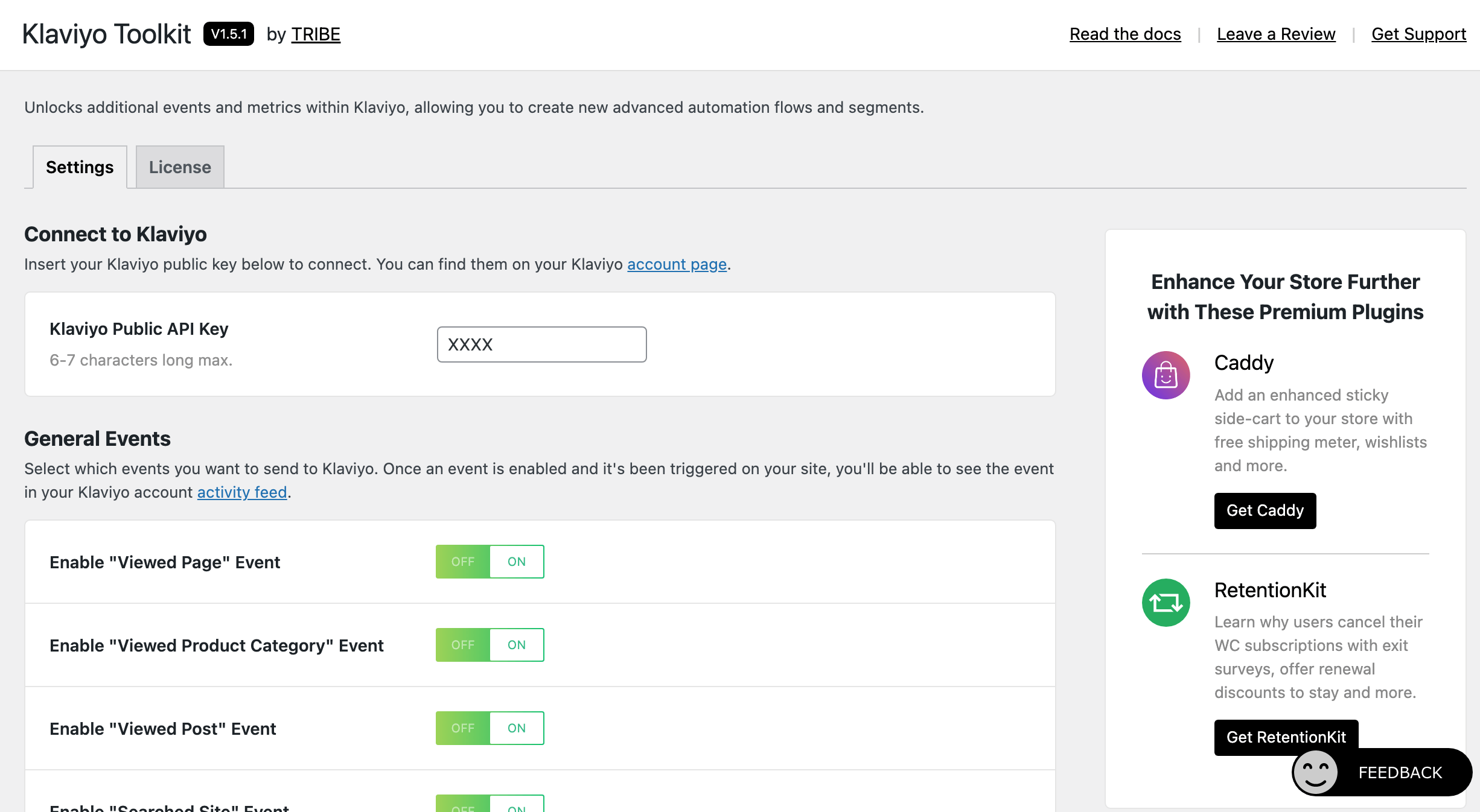Discover the Clavico Toolkit, featuring expanded events in the Americas, empowering you with Clavio to create advanced automated workflows and segments. Consult the comprehensive documentation, leave a detailed review, and access robust support to further enhance your store with premium plugins like Caddy and Retention Kit. Connect seamlessly to Clavio via the Clavio Public API, and ensure compatibility by enabling general events. Customize your tracking preferences with options to enable or disable viewed page, viewed product category, and viewed post events for a tailored integration experience.